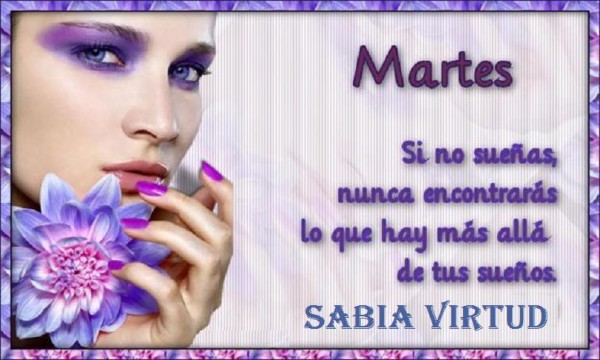The image appears to be a rectangular advertisement or business card, predominantly in shades of lavender, purple, pink, and blue. A woman occupies the upper left portion of the image, gazing seriously at the camera. Her face is adorned with extensive purple eye shadow that extends out from her eyes, both on the upper and lower lids, creating a striking, dramatic effect. She has pink lipstick and purple nail polish on her fuchsia-colored nails, one of which is holding a large purple flower near her face, adding to the sense of elegance and sophistication.

The woman's hand is curved towards her chin but does not touch her lips. Despite the close-up framing that excludes her hair and ear, her right cheek and left eye are clearly visible. She's situated in front of a lavender and white gradient background that hints at a wallpaper-like pattern with vertical stripes.

Surrounding the image is a decorative border, transitioning from purple shades at the top to pink floral patterns at the bottom, maintaining a purple-pink gradient on the right side.

On the right, there is a block of text in Spanish. At the top, in dark purple font, the word "MARTES" stands out. Below it, another message is written in slightly lighter purple, reading: "Si no sueñas nunca encontrarás lo que hay más allá de tus sueños." This is followed by the phrase "Sabia Virtud" in a blueish-green font.

Overall, the advertisement exudes a sense of beauty and elegance, likely intended for a nail salon or beauty-related service, emphasizing the woman's makeup and manicure.